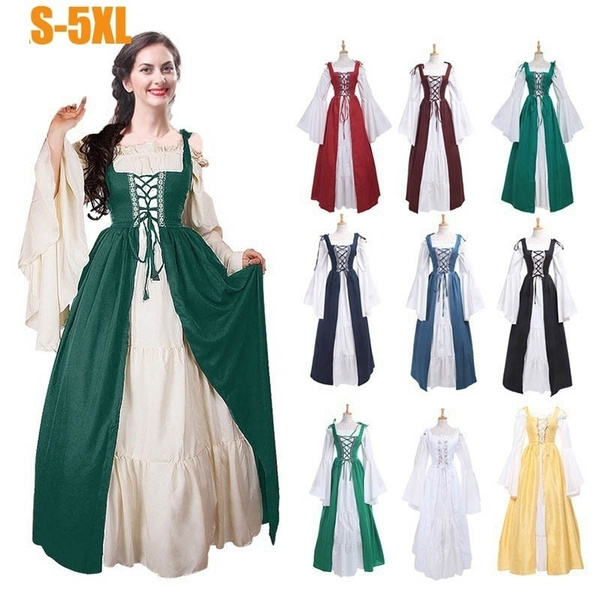This advertisement image features a woman with long, brown braided hair, dressed in a distinctive maid-style outfit with a cinched waist, a corset front, and floor-length draped sleeves. The dress showcased is notably green and white, with the green fabric being the part that varies in the different color options. She is smiling and wearing red lipstick, with her right hand pointing towards the top left of the image where bold, orange text reads "S-5XL," indicating the available sizes from small to five extra-large. The right side of the image displays the same dress design in nine different color variations arranged in three rows of three: red, burgundy, green, navy blue, black, blue, light green, white, and yellow. The background is white, making the colorful dresses and the detailed model on the left the focal points of the advertisement.